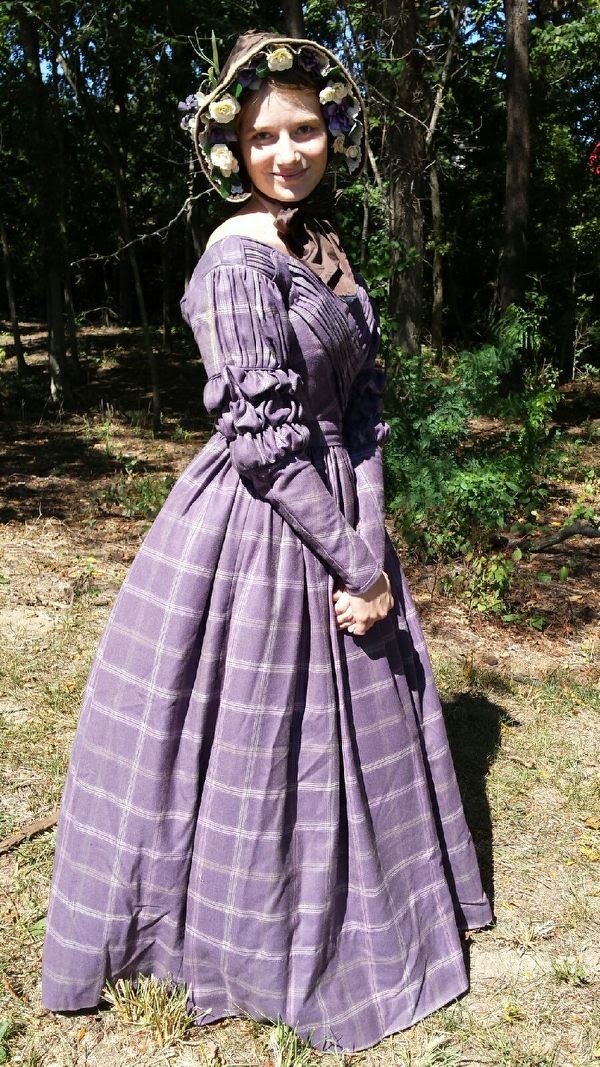In this sunlit outdoor photograph, a woman stands on a grassy area, framed by lush, green trees and a bush. She is dressed in a light purple, floor-length, period costume with puffy, ruffled sleeves that extend from the shoulder to the elbow. The skirt of her dress is adorned with horizontal lines and slightly drags on the ground. She wears a hat decorated with white roses lining the brim, adding a touch of elegance reminiscent of a bygone era. Smiling warmly and looking directly at the camera, she crosses her arms at her waist, evoking a sense of serene confidence. The scene is vibrant with natural greenery, though patches of the grass appear somewhat dry, emphasizing the authenticity of the outdoor setting.